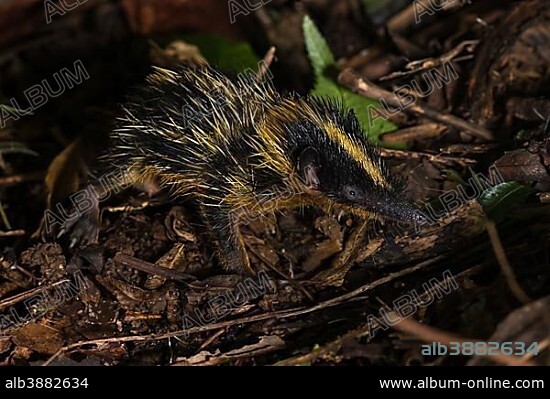This is a photograph of a small, mole-like rodent with a long, pointy snout and a teeny eye, situated on a moist forest floor at night. The rodent features a distinctive mix of black and yellow fur, with whitish spikes that glimmer slightly as if wet. The animal is facing slightly to the right but with its snout pointing more directly at the camera. It is perched on a pile of broken twigs and leaves, with a few green leaves visible amongst the wood. The image is watermarked multiple times with the word "album" embossed across it, and at the bottom, a thin black border holds the labeling "ALB3882634" on the left and the website "www.album-online.com" on the right. The scene captures a detailed view of the rodent in its natural forest habitat, underlining the damp, rich texture of the environment.